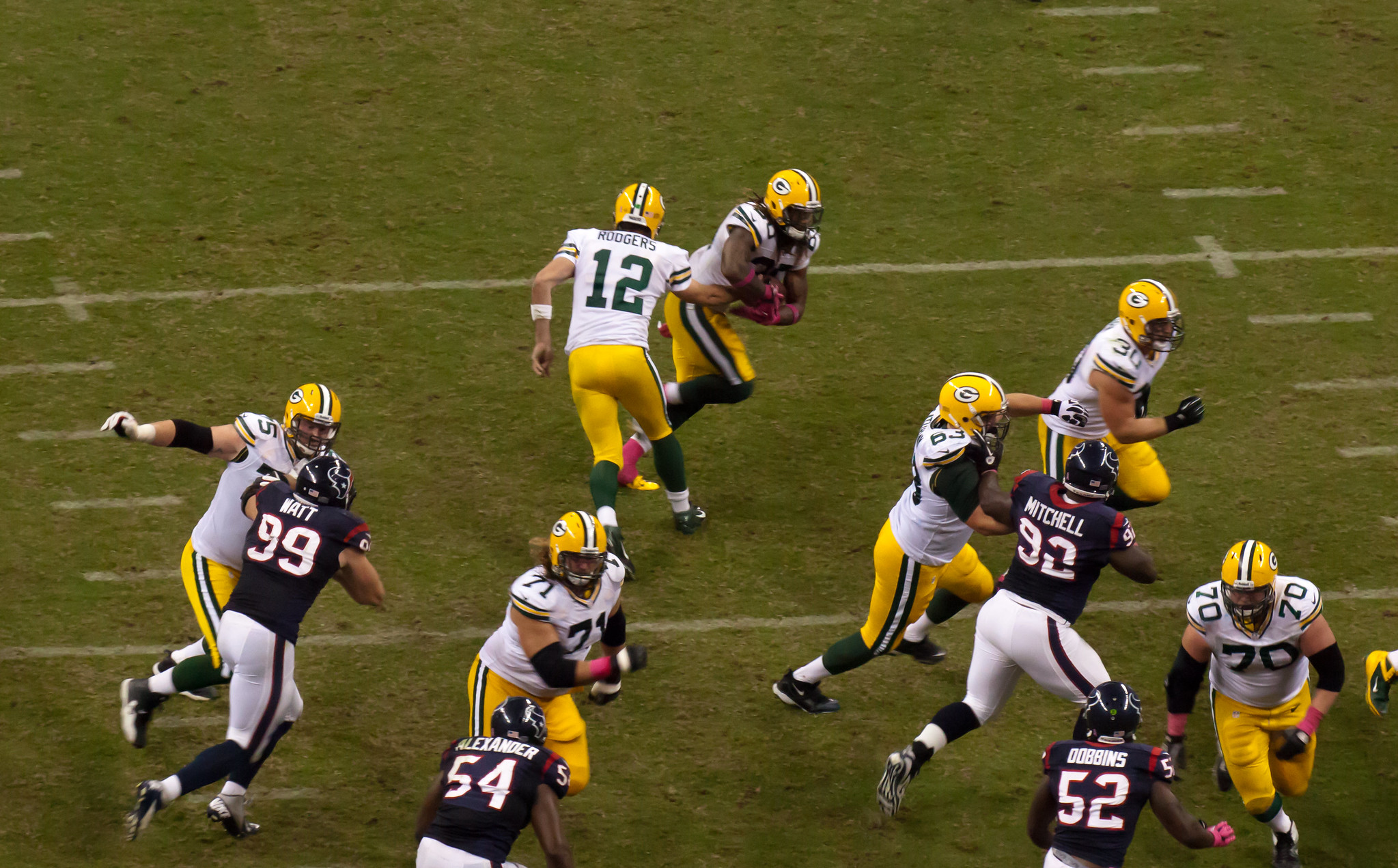The square photograph captures an intense moment in an American football game between the Green Bay Packers and the Houston Texans. The field is marked by horizontal yard lines and vertical hash marks, emphasizing its gridiron structure. The Packers, identifiable by their home white tops, gold pants, and green accents, dominate the action. Aaron Rodgers is in the midst of handing off the ball to a running back who charges to his left, flanked by six blockers. In opposition, four Houston Texans, dressed in dark jerseys with white pants and dark piping, scramble to tackle the runner. The scene is set during the daytime, as evidenced by the players' shadows stretching across the green grass. The players primarily occupy the lower half of the image, with only two venturing into the upper half, which remains largely as negative space.